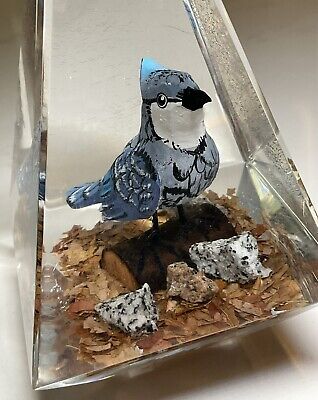The photograph captures a detailed sculpture of a blue jay, meticulously carved with a blue body, black feathers, and a black beak, showcasing a distinct white patch underneath its beak. The bird is perched on small legs atop a brown, cut wooden log, surrounded by wood shavings. In front of the log, three distinct pieces of quartz—two white and one light brown—rest artistically. This entire arrangement is encased within a clear plexiglass box that narrows towards the top, resembling a pyramid. The box provides a clear view of the intricate sculpture against a white background.